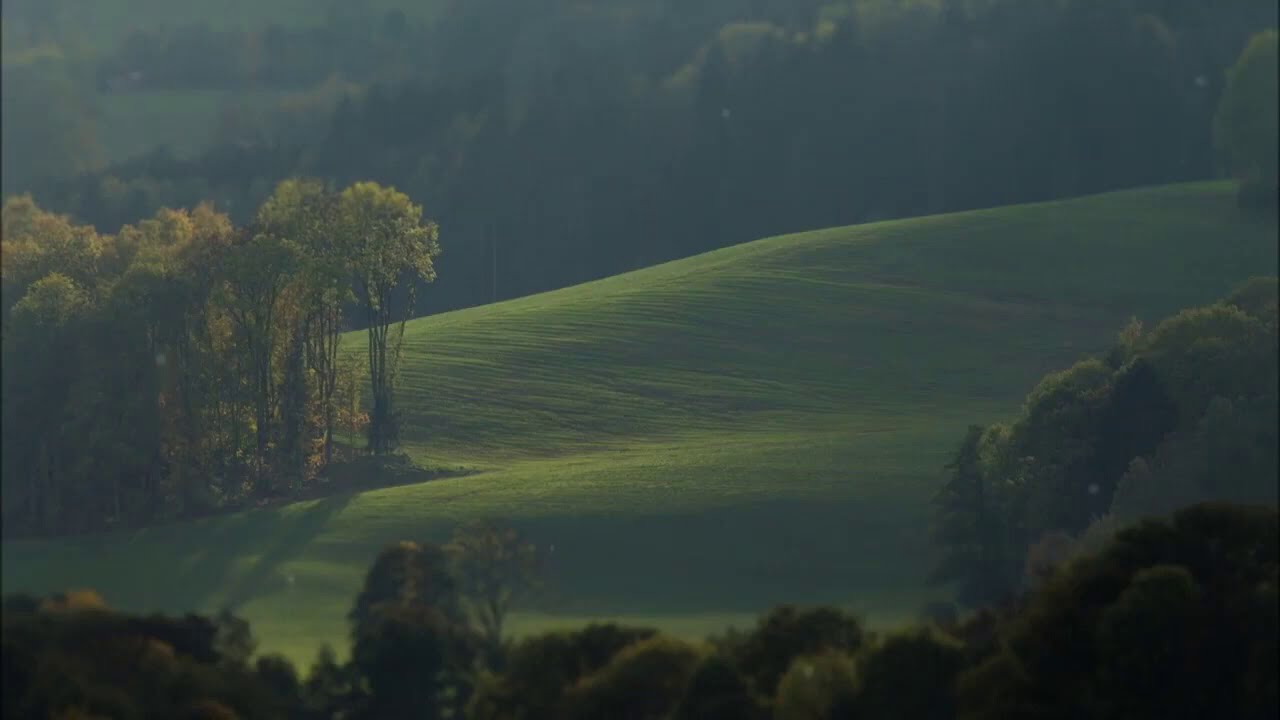The image is a breathtakingly detailed depiction of a nature setting, resembling either a hyper-realistic painting or a professionally captured photograph. The scene is set in a vast landscape that could be a golf course, valley, or meadow, characterized by lush, rolling green hills. It's likely captured in the late afternoon, shortly before dusk. The hills are blanketed with meticulously manicured grass, and sunlight spills across the landscape, casting glints and illuminating parts of the scene with soft yellow light.

The foreground features a diverse array of trees with dark green foliage, some showing early signs of fall with yellow and orange accents. These trees, along with scattered bushes, frame the lower part of the image, adding depth and a sense of serenity. To the left, a notable group of trees with brown stems is partially lit by the sun. Further into the background, additional hills and mountains covered in dense trees and bushes appear slightly hazy and blurred, giving the image a sense of distance and tranquility.

The photo's palette includes various shades of green, complemented by touches of black, brown, white, and the warm tones of yellow and orange. Despite its vividness, the image retains a certain stillness, devoid of people, text, or water, capturing the unspoiled beauty of nature. The collection of trees and expansive grassy areas come together to create a serene and captivating scene.